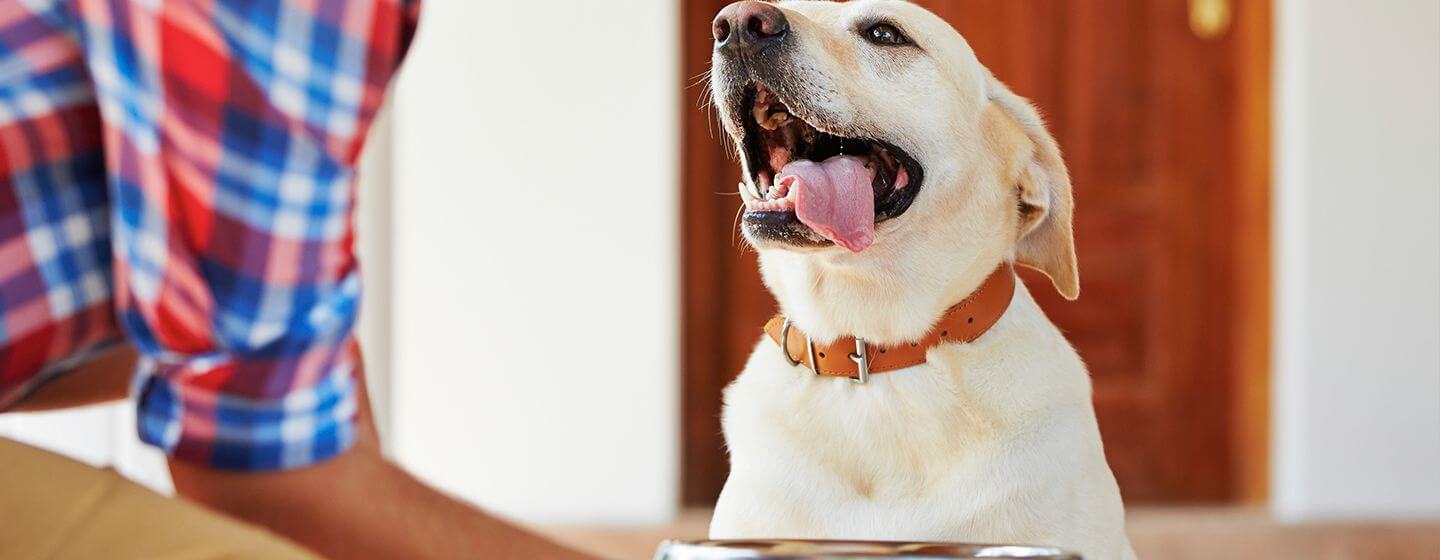The image features a happy, beige Labrador dog with a brown collar and a pink nose, its tongue playfully hanging out. The dog appears to be an adult rather than a puppy and has black eyes. To the left, partially visible, is a man dressed in a blue and red plaid shirt and tan khakis. He seems to be petting and paying attention to the dog. In the indoor setting, there are white walls and a wooden door with a gold doorknob in the background. A silver bowl, likely for the dog's food or water, sits in front of the dog, further enhancing the cozy domestic scene.